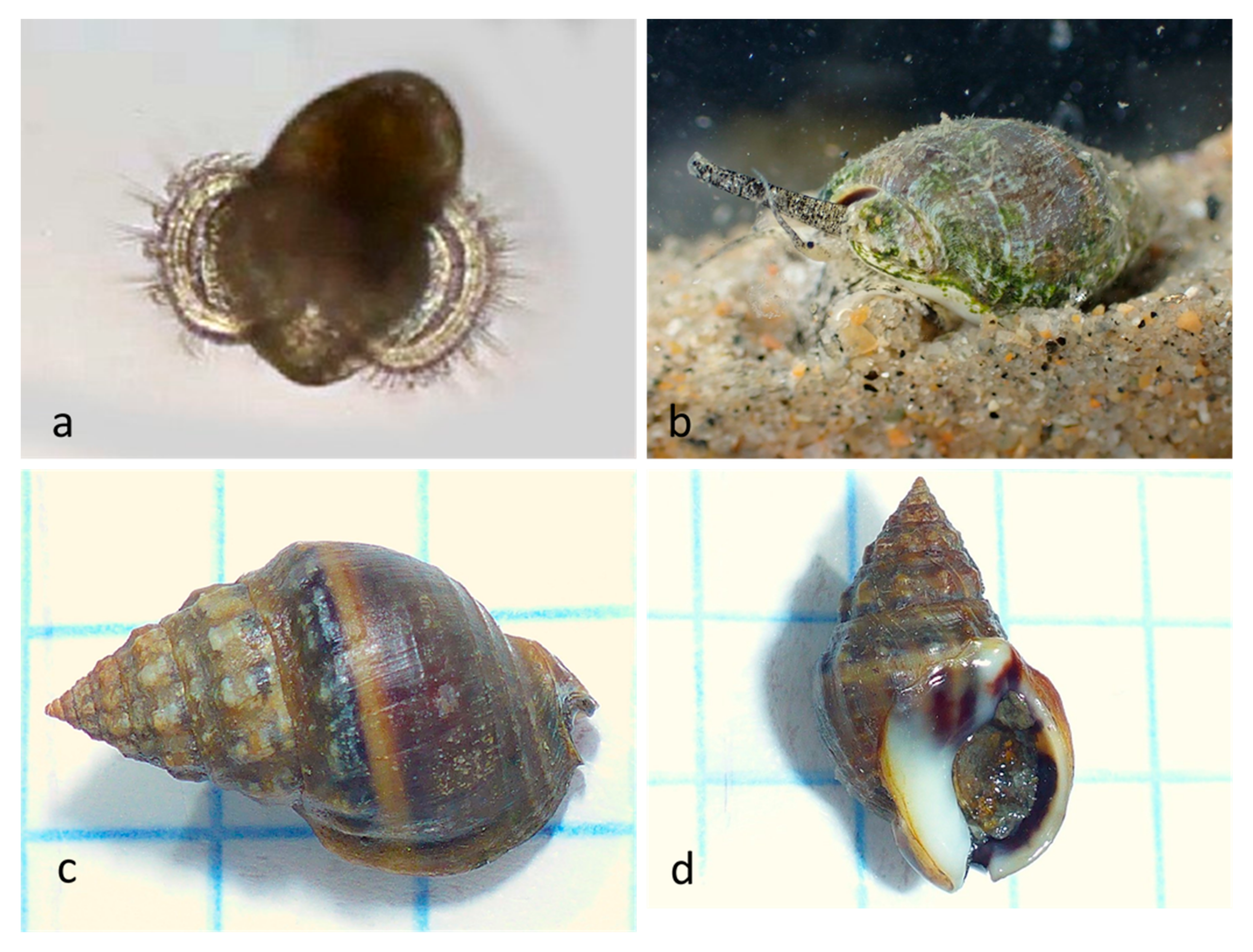The image consists of a collage of four labeled quadrants (A, B, C, D), each depicting various perspectives of snail shells against a predominantly white background with blue squares.

- **A** (top left): An enlarged, microscopic view showing a small brown speck with two circular shapes on each side—possibly a baby snail or a different organism.
- **B** (top right): A close-up of a snail in a greenish-brown shell, partially submerged underwater with visible sand and small rocks, displaying a protruding tentacle or antenna.
- **C** (bottom left): The exterior of a pointy snail shell, featuring distinct brown and yellow stripes, set against the white and blue gridded background.
- **D** (bottom right): The underside of a similar striped shell, turned upside down to reveal the interior, which appears to contain a dark, goopy substance, also on the same gridded background.

These images collectively showcase different angles and close-ups of what seems to be the same or similar snail shells, highlighting various details both inside and outside the shells.